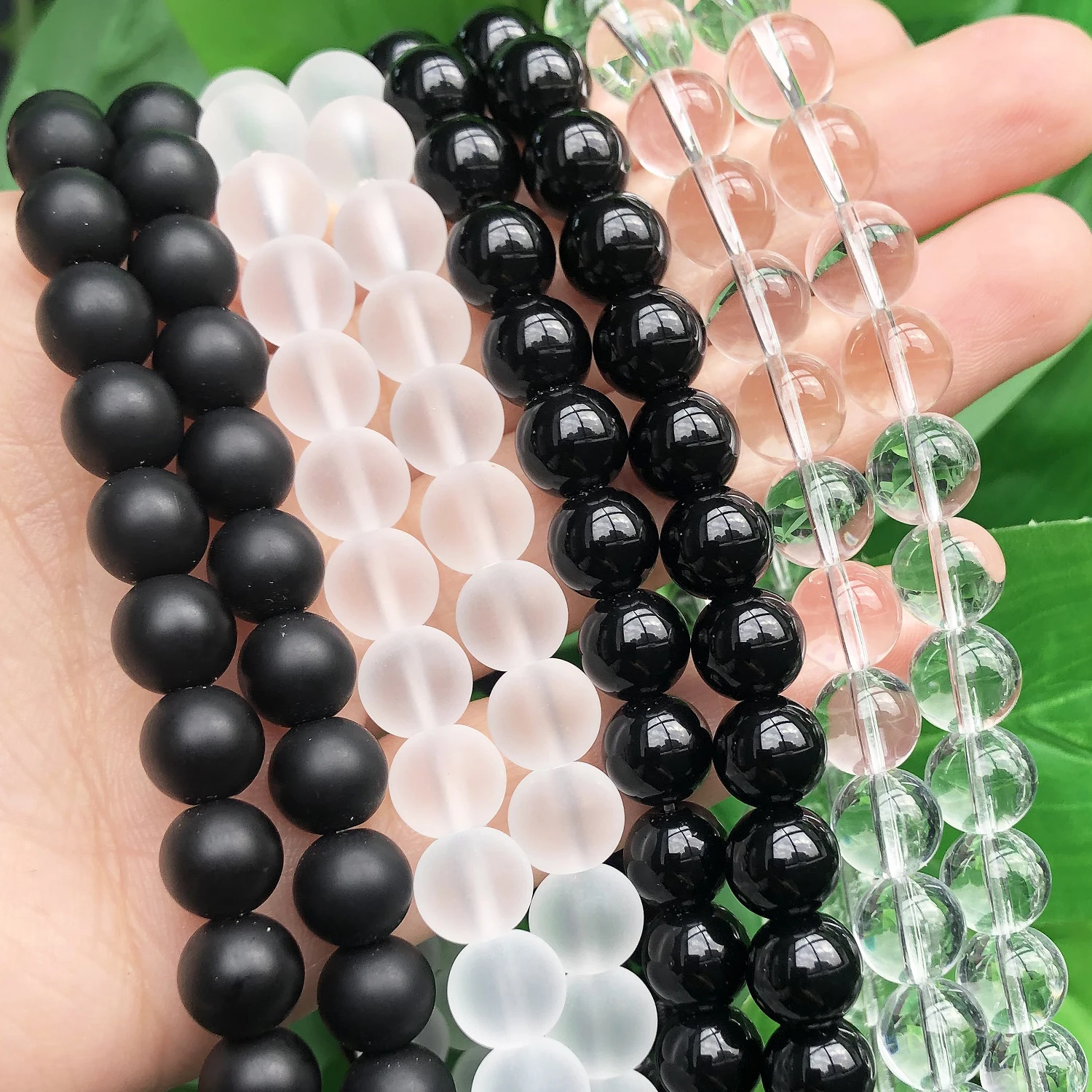In this close-up photograph, a hand is prominently featured in front of a softly blurred green background that appears to be leafy foliage, showcasing various shades of green. The hand, held palm up and fingers extended to the upper right, grips eight strands of beads, which run horizontally across the palm. Beginning from the left, there are two strands of matte black beads, possibly a single strand wrapped twice, characterized by their round and uniform shape. Adjacent to these are two strands of somewhat translucent, white beads, where the cord running through them is faintly visible. Following these are two strands of shiny, glossy black beads, exuding a marble-like sheen. Finally, on the far right, two strands of crystal clear beads complete the arrangement, their transparency revealing the cord inside.